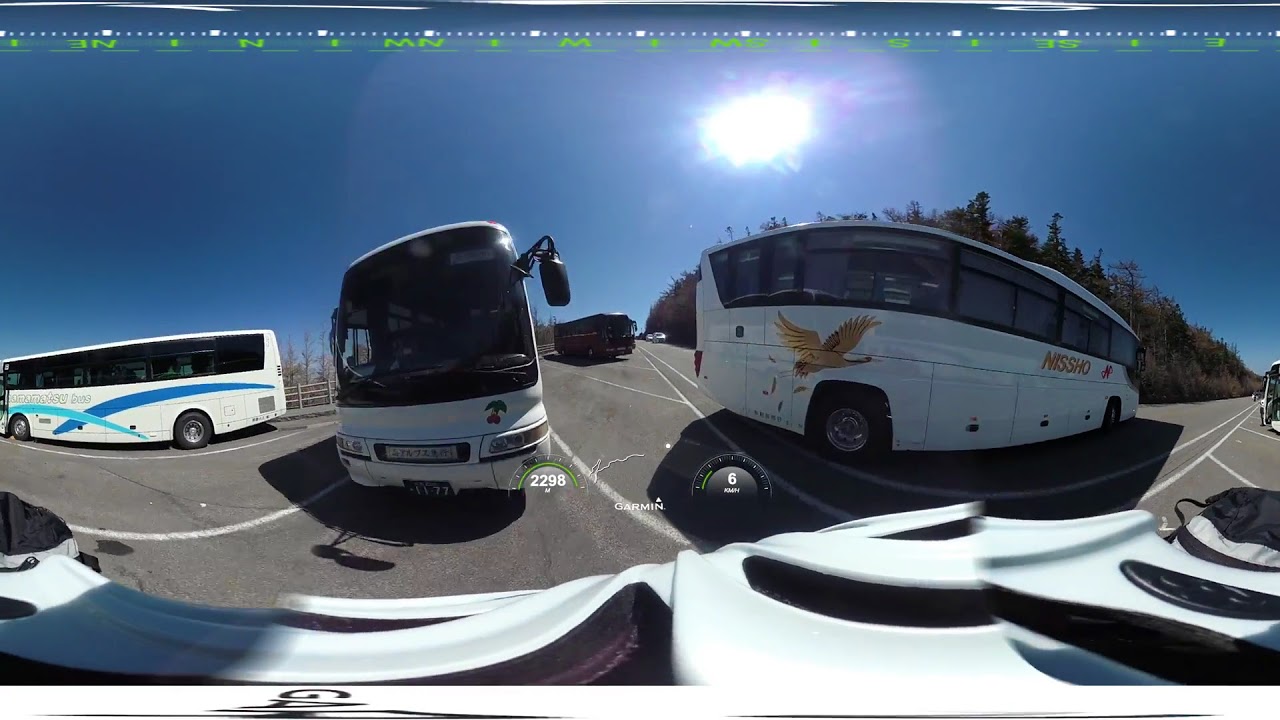This panoramic 360-degree image captures an outdoor parking lot with gray asphalt and white lines for bus parking spaces. Three white buses are prominently parked. The bus on the right features the name "NISSHO" along with a gold-colored eagle image and appears somewhat warped due to the panoramic view. The bus in the center is facing head-on, showcasing its large windshield and a distorted view at the bottom that might be the hood of another bus. The left bus displays two overlapping stripes in teal and blue, resembling Nike swooshes, with unreadable text over them. Additional details include a small dial labeled "2298 Garmin 6" to the right of the distorted foreground object. In the background, a wooded hill and a bright blue sky with a distorted sun are visible, hinting at the image being taken in an Asian country, inferred from a bus license plate and the names on the buses. Farther in the distance, you can also spot some cars.